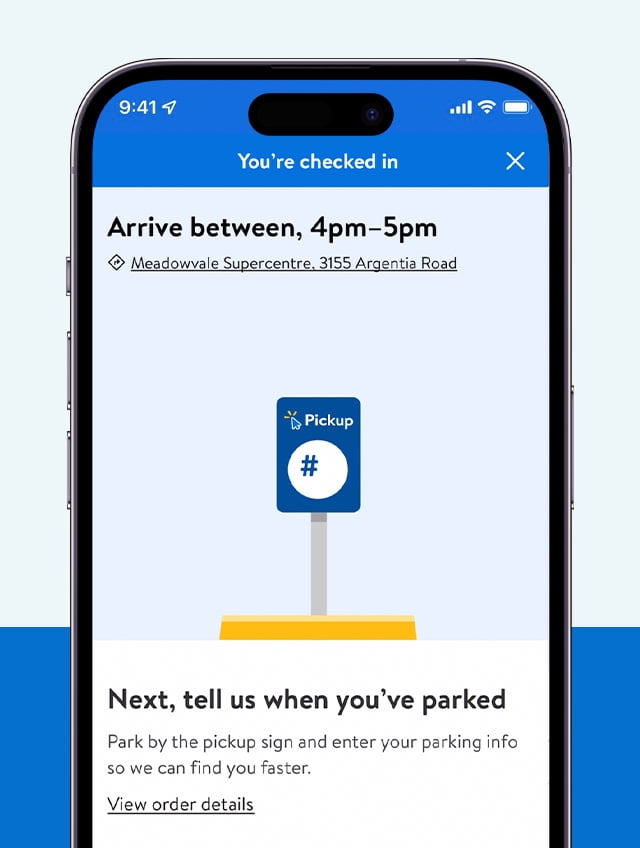The image depicts a detailed mock-up of a person interacting with a mobile application. The scene showcases the upper part of an iPhone, clearly indicating it is a screenshot taken from the device. At the top, the status bar is visible, showing the time as 9:41, full Wi-Fi signal, and 100% battery life.

The app interface prominently displays a notification stating, "You're checked in," with an "X" close icon to the right for dismissal. Below this, in white text, it instructs the user to "Arrive between 4 p.m. and 5 p.m." at "Meadowvale Supercenter, 3155 Argentina Road."

Central to the interface is a graphic element featuring a blue sign on a gray post beside a yellow painted curb. The sign bears the word "Pickup" and includes a circular icon with a pound sign (#) situated in the bottom third of the sign. A mouse pointer icon, emitting three yellow flares to indicate a click, is positioned near the text: "Next, tell us when you've parked. Park by the pickup sign and enter your parking info so we can find you faster." Below this directive, an underlined option reads "View order details."

In the background of the image, outside the phone's screen, there is a noticeable bright blue bar peeking from both sides at the bottom of the image, contrasting with the white area above. The edges of the phone and its buttons are also discernible, adding realism to the mock-up.